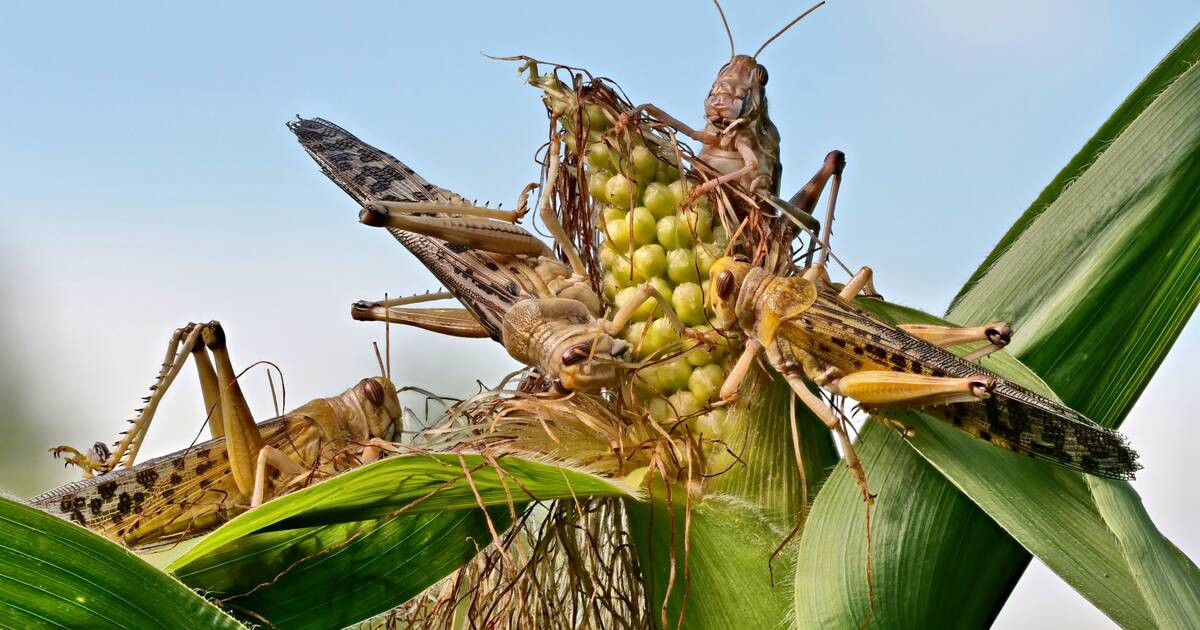The photograph showcases an ear of corn that is still green and not yet ripe, with large, green leaves that have been pulled back to expose the yellow kernels. The corn is infested with four locusts that are busy devouring the kernels. Each locust, which closely resembles a grasshopper, has six legs with two large, bent hind legs adapted for hopping. They sport a yellowish-beige coloration with black spots, and have beady brown eyes and beige wings. The locusts are positioned in various manners around the corn: one locust is bent downward biting into the corn, another is angled toward the top right standing on a husk, a third is directed toward the top left and consuming the corn, while the fourth appears from behind the corn, standing upright and wrapping its legs around it. The background of the image features a slightly blurry, light blue sky with faint hints of clouds, indicating that the photograph was taken outdoors during the daytime. The presence of potential additional locusts is hinted at by the sight of distinctive legs or antennae extending from behind the ear of corn.